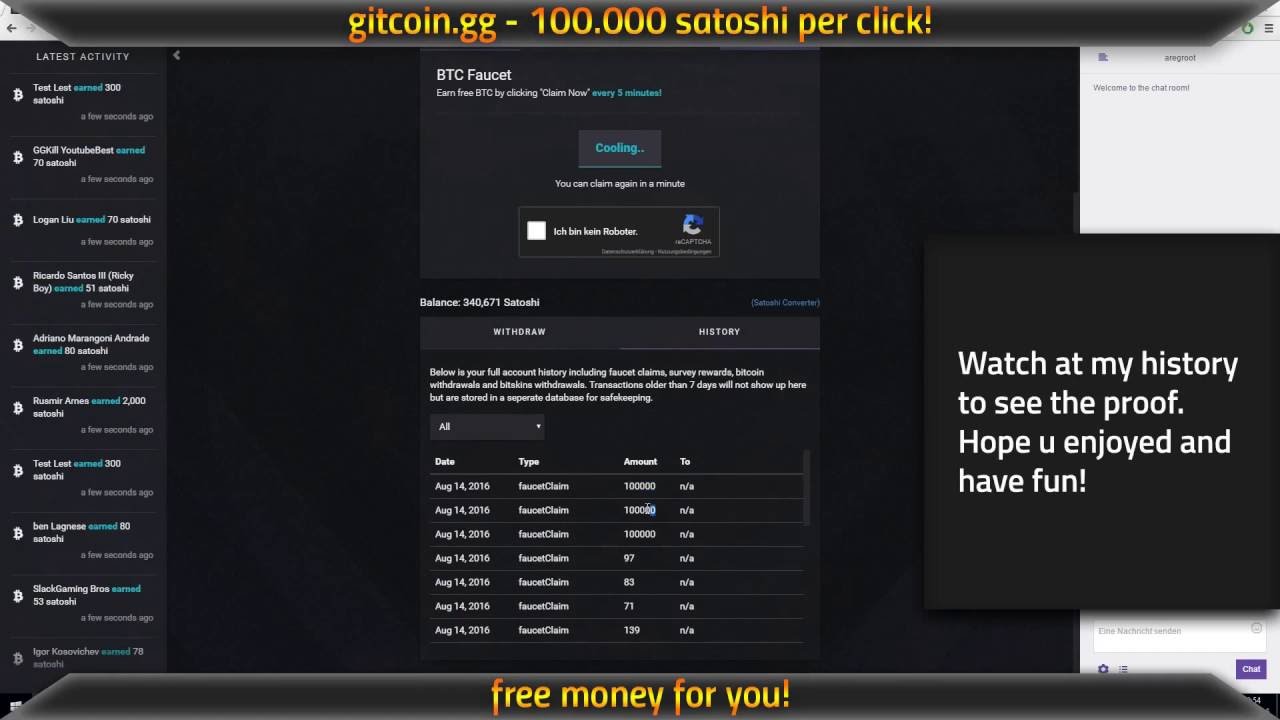The screenshot displays a section of the website "getcoin.gg", specifically showcasing a Bitcoin faucet that rewards users with Satoshis for their activities. 

At the top, the banner prominently reads "getcoin.gg - 100000 Satoshi per click". The site's name, as displayed, uses the spelling "g-i-t-c-o-i-n".

On the left side, there's a navigational panel listing recent user activities in small text. Each entry includes a username and the amount of Satoshis earned recently. For example:
- "ggkillyoutubebest earned 70 Satoshi a few seconds ago"
- "Logan Liu earned 70 Satoshi a few seconds ago"
- "Rusmarmia earned 2,000 Satoshi a few seconds ago"

The main content area, centered on the page, features a large heading "BTC Faucet". The instructions below prompt users to "earn free BTC by clicking claim now every five minutes". Beneath this is an area currently inactive with the text "cooling, you can claim again in a minute". 

There is also a CAPTCHA verification box labeled "Ich bin kein Roboter" (translating to "I am not a robot" in German) reaffirming user authenticity. Below this, the balance is displayed as "340,671 Satoshi".

Two additional tabs, "Withdraw" and "History", are visible below the balance; the "History" tab is currently selected. This section provides a detailed transaction history where each row includes:
- Date (all set as August 14, 2016)
- Type (all listed as "faucet claim")
- Amount (ranging between 71 and 139 Satoshi)
- Status (not applicable, marked as "N/A")

To the right, a black notification box overlays part of the chat area with the message, "Watch my history to see the proof, hope you enjoyed and have fun." The chat area itself is light grey, facilitating user interactions. 

Finally, at the bottom of the page, there's a bright ribbon that reads "Free money for you!" equipped with an exclamation point, encouraging further engagement with the site.

This descriptive caption offers a meticulous overview of the webpage, illustrating both its functional and interactive elements in detail.